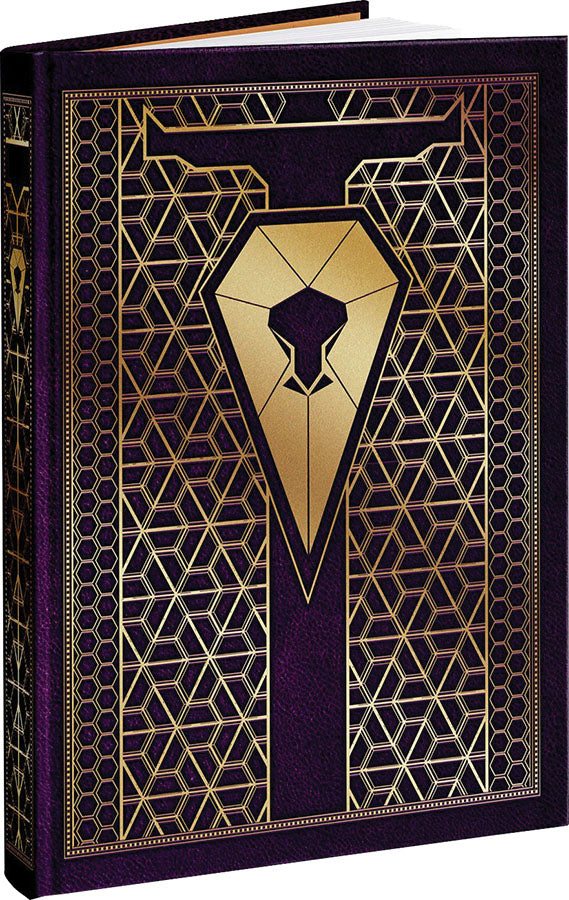This is a photograph of a hardcover book standing upright and partially open, revealing its pristine white pages. The book is bound in a dark purple cover adorned with an intricate gold geometric design that resembles a science fiction aesthetic. Central to the design is a diamond-shaped shield featuring an abstract, superhero-like head. The cover's elaborate gilt pattern extends in a web-like fashion across both sides of the book, adding to its mysterious appearance. Despite its eye-catching design, the book lacks any visible title, author's name, or other identifying text, suggesting it could be anything from a personal diary to a religious or cult-like tome. The cover has no slip cover, emphasizing its elegant and somewhat enigmatic presentation.